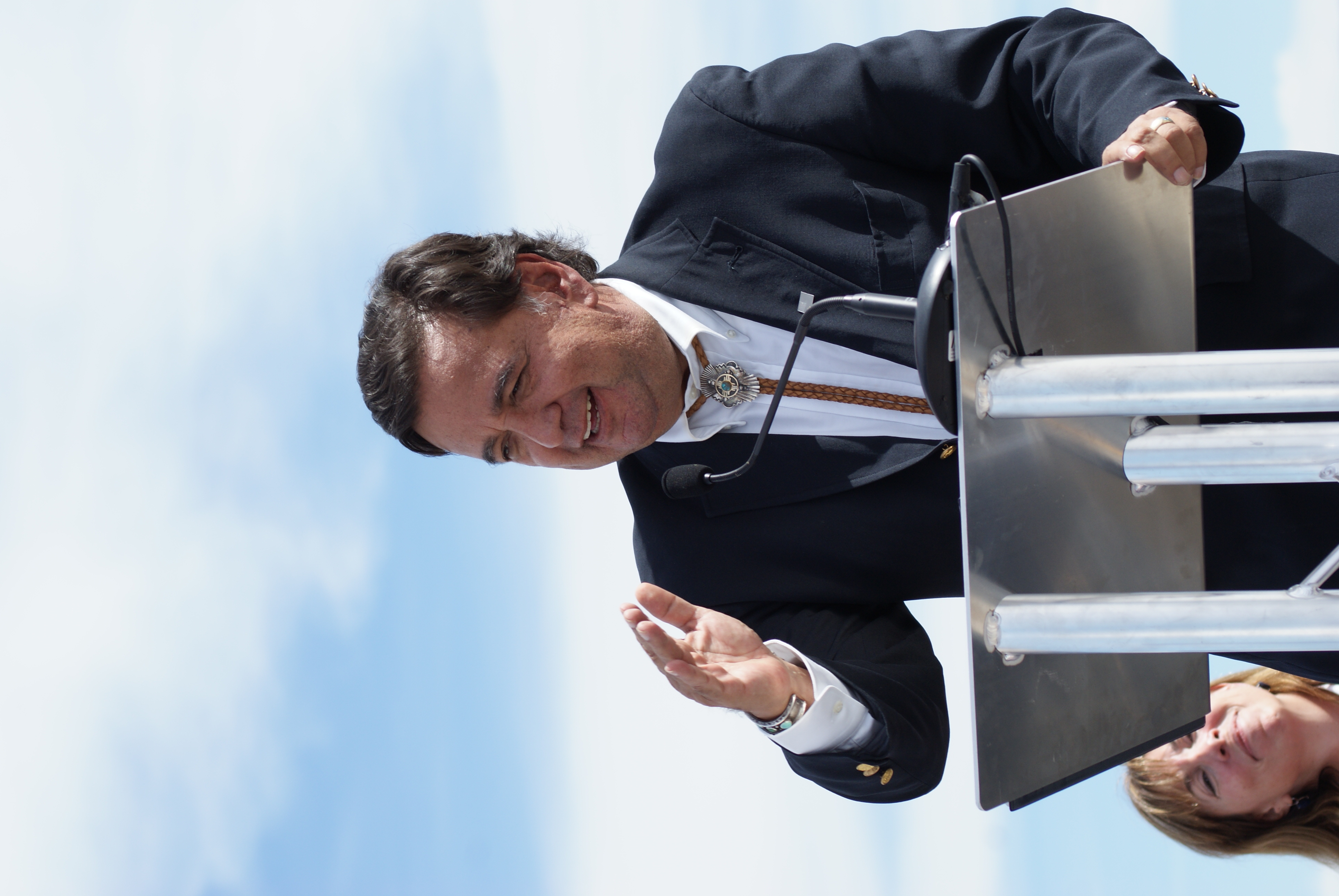This image is rotated incorrectly, with the bottom on the right side and the top on the left side. It depicts a man in a black business coat with a white button-up shirt, turned-down collar, and a leather braid with a silver brooch around his neck. He is standing behind a metal podium composed of three blue rods welded to a flat metal surface. On this surface rests a black plastic base holding a built-in black microphone. A wire from the base wraps around one of the metal rods. The man has a silver bangle on his right arm, which is raised, and appears to be giving a speech. A partially cloudy blue sky suggests the event is outdoors. In the background, a woman is partially visible, with only her head showing in the lower left-hand corner of the image. The entire scene is captured sideways, making the vertical elements appear horizontal.